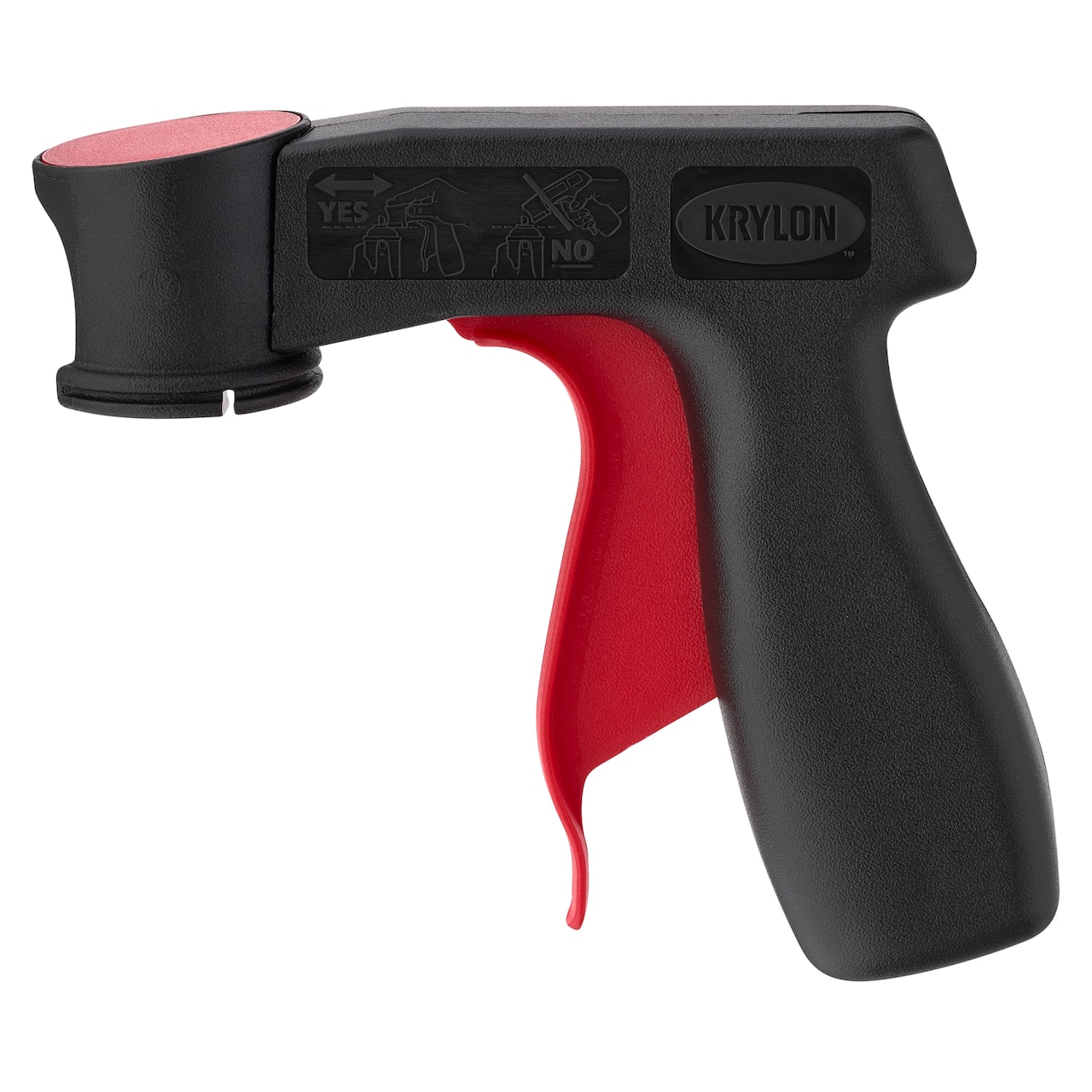This studio-shot image showcases a sleek spraying device, primarily composed of smooth, flat black plastic, designed in a gun-like shape with a long handle and a barrel pointing forward. The standout feature is the wide red trigger, which spans over half the length of the handle, providing an ergonomic design. The device, branded by Krylon, has its logo prominently displayed in an oval shape near the instructions. These instructions, etched into the side, include a diagram demonstrating the correct (marked "yes") and incorrect (marked "no") ways to use the tool. A small red circle, seen at the front of the barrel, adds a distinctive touch to the otherwise black device. The overall presentation of the tool, against a plain white background, highlights its functional design and user-friendly features.